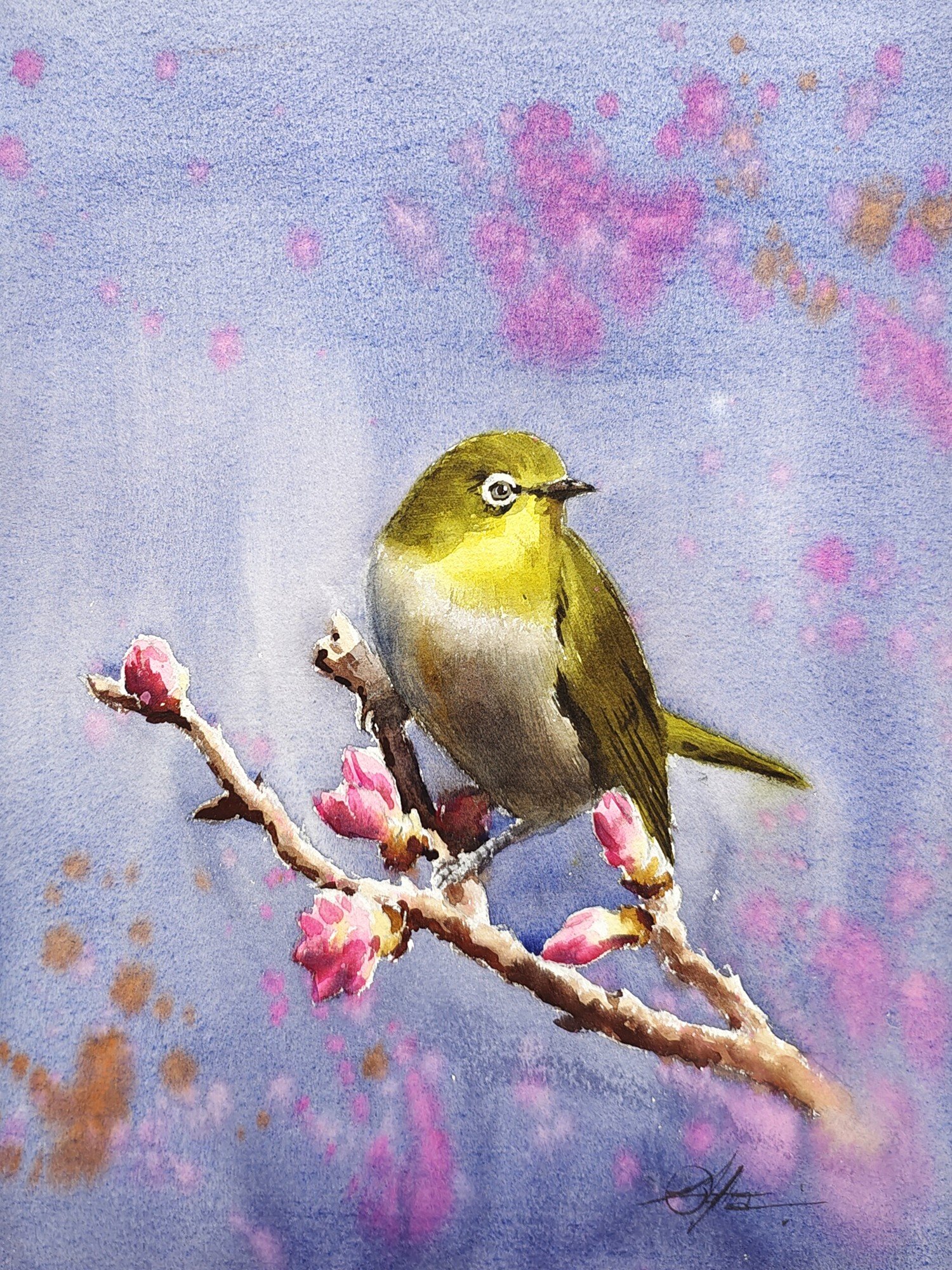The painting features a delicate, light blue background with subtle splotches of violet and light brown scattered throughout. In the center, a bird with golden plumage on its head, wings, and tail perches gracefully on a light brown branch adorned with budding pink and violet flowers. The bird, which has a creamy white breast, small beak, and gray eyes, looks to the right, revealing only one eye. The intricate branch stretches diagonally from the lower right to the upper left of the image, intersecting areas with soft pink and tan patches. In the lower right corner, there is an artist's signature, though it remains unreadable. The composition is harmonious, blending gentle hues and delicate details to create an enchanting, serene scene.